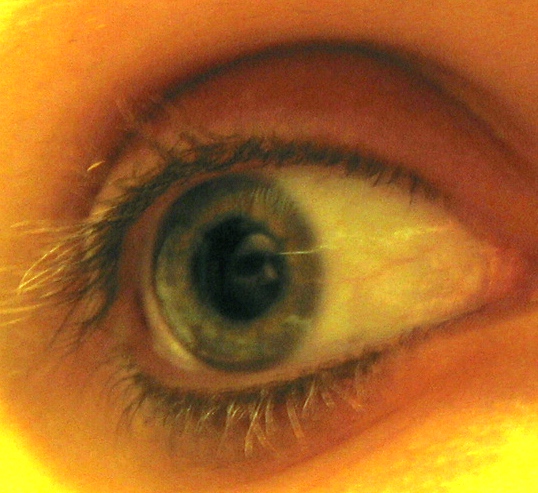This square-shaped photograph captures a close-up of a person's eye with striking detail. The eye, belonging to a person with blue corneas, is the primary focus, showing delicate features such as long, thick eyelashes both on the top and bottom without any makeup. The image quality suggests it was taken with an older camera, giving it a vintage feel. The eye appears healthy with visible veins in the sclera (white part of the eye). The iris is prominently on the left, indicating the person is looking slightly to the left. A fascinating aspect of the image is the reflection in the pupil; it shows a partial reflection of another face, seemingly a white person, with visible features including their eye, nose, and cheekbone. This reflection, which includes a hint of dark hair, adds an element of intrigue to the photograph. The detailed features of the eye, including the precise depiction of the eyelashes and the reflected face, make this image both captivating and slightly eerie.